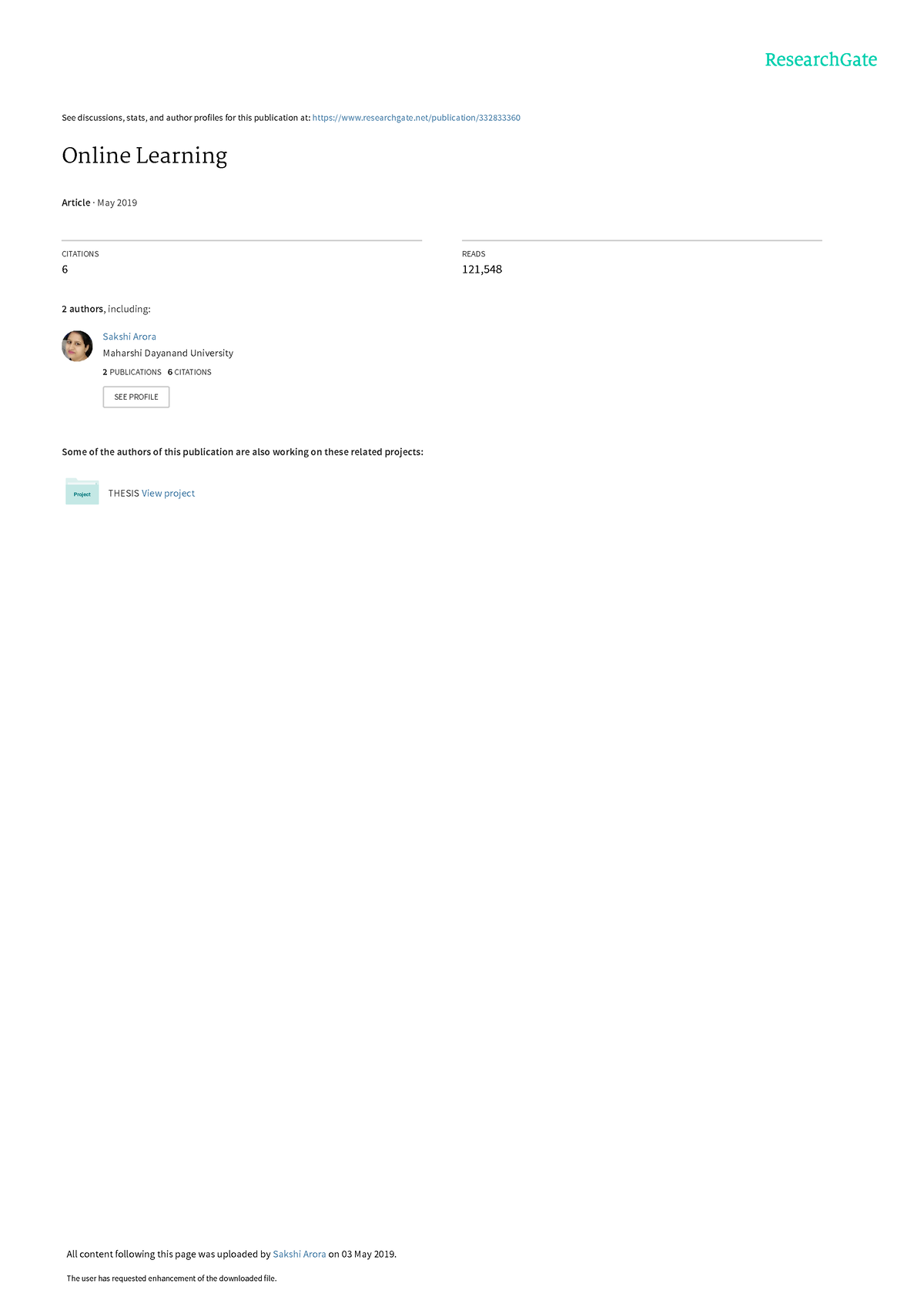This screenshot, taken from a ResearchGate webpage, showcases various elements related to a publication. At the top of the screen, there's a navigational bar stating "See discussions, stats, and author profiles for this publication at" followed by a clickable URL in blue text: "http://www.researchgate.net/publication/[long blue number]". In the top right corner, the ResearchGate logo is displayed in a teal green color.

Centered on the page, the title "Online Learning" appears in prominent black print. Directly below the title, in smaller print, it reads "Article - May 2019".

A gray line separates the title area from additional publication metrics: 

- "Citations: 6" positioned on the left.
- "Reads: 121,448" on the right, divided by another faint gray line.

Further down, the publication lists two authors, highlighting a profile picture of a woman who appears to be of Indian descent. The detailed information next to the profile includes her name, "Sakshi Arora", and affiliation, "Maharshi Dayanand University". It mentions she has two publications and six citations. 

Towards the bottom, there's a small teal-colored file folder icon labeled "Thesis," adjacent to a clickable link "View Project."